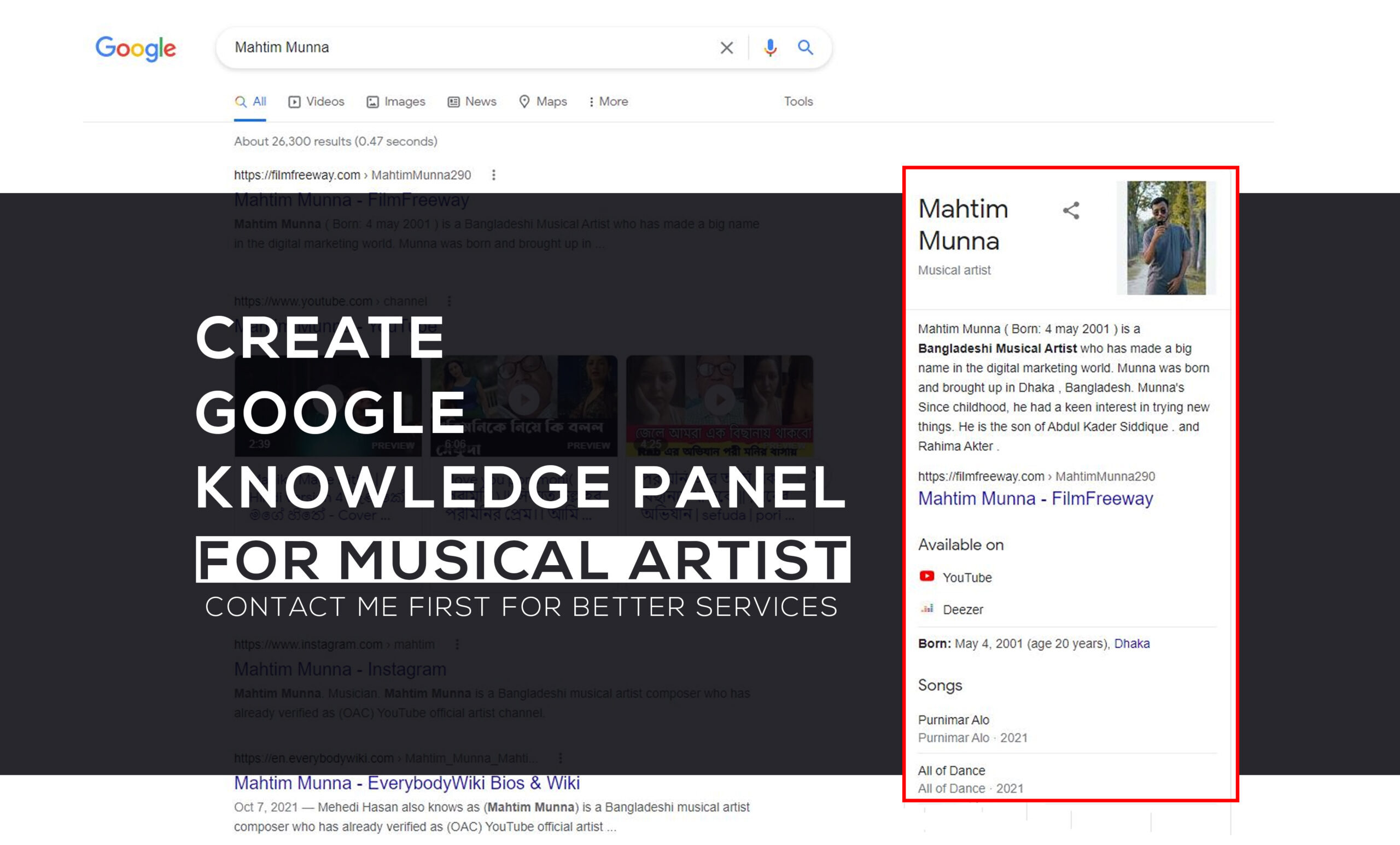The image depicts a Google search results page, where the search term "Matamuna" has been entered into the search bar. The page displays options for different types of search results: All, Videos, Images, News, Maps, More, and Tools. Below these options, it shows that there are approximately 26,300 results found in 0.47 seconds.

In the center of the page, a prominent black box obscures part of the search results. Inside this box, white capital letters indicate "CREATE GOOGLE KNOWLEDGE PANEL" and an additional message addressing musical artists, stating "Contact me first for better services."

To the right side of the screen, a white rectangular box with a red border partially covers the black box. This white box provides a brief biography of Matamuna. It states that Matamuna was born in May 2001 and identifies him as a Bangladeshi music artist who has achieved significant recognition in the digital marketing realm. The text mentions that Matamuna's mother was born and raised in Bangladesh and that he (Matamuna) has always been keen on exploring new ventures. The remaining text appears too blurry to read clearly.